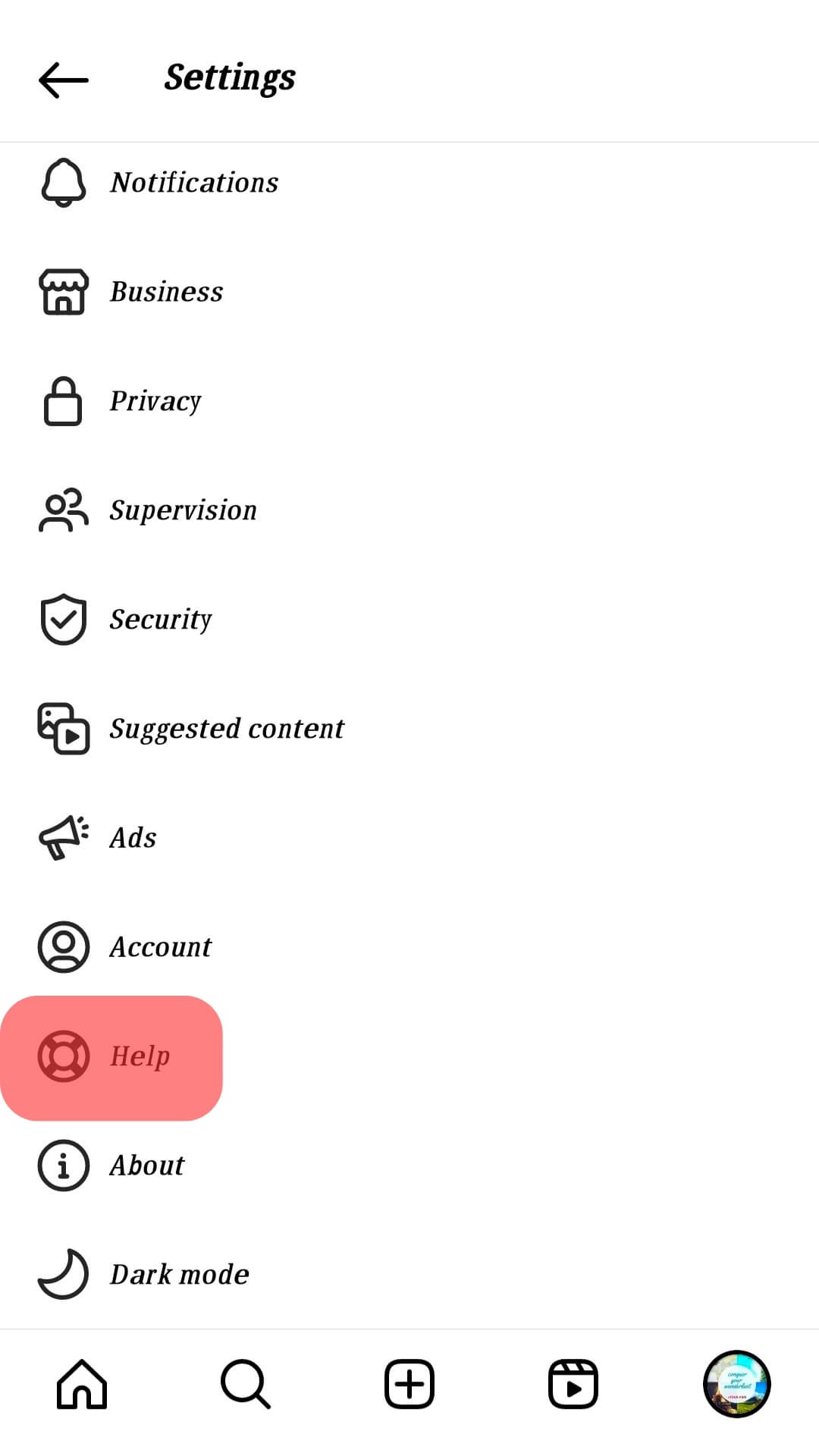The image showcases a settings panel with a clean, white background. At the top, there's an arrow pointing to the left, next to the word "Settings" in bold, italicized font. Below this, a thin grey line separates the header from the rest of the panel.

The main section of the panel consists of a list of options, each with a corresponding icon, all rendered in black and white. The first item is "Notifications," accompanied by a bell icon. Following that is "Business," paired with a hut icon. 

Next, the "Privacy" option is represented by a lock icon, and "Supervision" has two person icons. Subsequently, "Security" features a shield with a checkmark, and "Suggested Content" is denoted by a play button over a photo icon.

"Ads" is marked by a megaphone icon, and "Account" has a circle with an outline of a person inside it. The "Help" option stands out with a big red bubble that encompasses both the word "Help" and its accompanying circular icon, which features a smaller circle with black rectangles on each diagonal corner.

After "Help," the list includes "About," identified by a circle with an 'i' inside it, and "Dark Mode," shown with a crescent moon icon. 

A thin grey line separates these options from a set of navigation buttons at the bottom of the panel: a house icon, a magnifying glass, a square with rounded corners and a plus sign in the middle, a movie frame with a play button, and a colorful circle, presumably a logo, dominated by blue and white hues.

This setup highlights various settings and options available in a user-friendly interface, with intuitive icons to guide navigation.